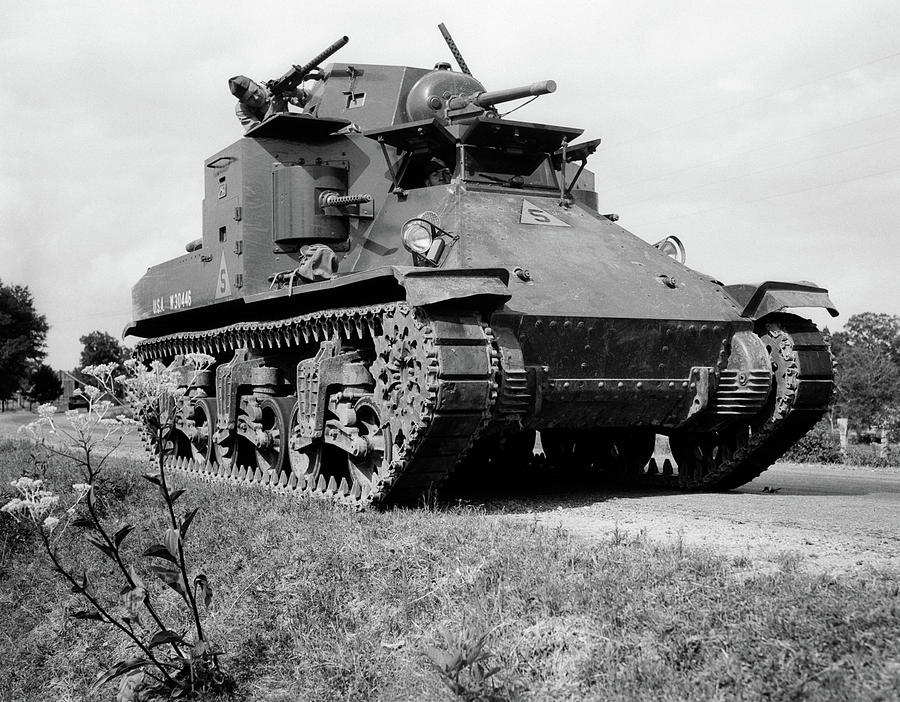The image features an old military tank in a black-and-white photograph, suggesting it might be from around the World War II era. The tank is navigating a dirt road that appears to slope down into a grassy ditch on the left. In this ditch, a few blooming flowers, possibly weeds, add a touch of detail. The road and surrounding area are framed by a number of trees, mainly in the background with some appearing on the right side. The overcast sky adds a somber atmosphere. 

A soldier or man in military attire is visible atop the tank, engaged with the main gun or turret, which is pointed slightly upwards. This person seems to be looking through the gun's sight, potentially preparing to fire. The tank features a long traction system with visible wheels and a distinctive white identifier on its left side, likely denoting "USAW30446" and featuring a triangle with the number 5 both on the left side and at the front. A faint fence can also be discerned in the background, adding another layer of context to this wartime scene.